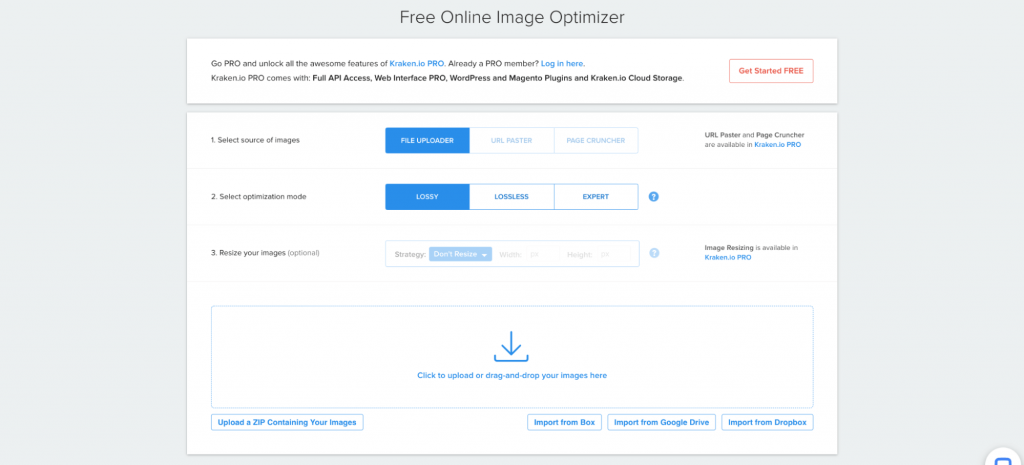On a gray background, this image prominently features the header "Free Online Image Optimizer" in a slightly darker gray font. Below this, there's a white rectangular box announcing "GoPro and unlock all the awesome features of Kraken.io Pro." A call to action for existing Pro members to log in is also included. 

The box highlights the benefits of Kraken.io Pro with a list in bold black font: "Full API Access, Web Interface Pro, WordPress and Magento Plugins, and Kraken.io Cloud Storage." A white button with red font encourages users to "Get started free."

Another white box beneath offers various options for image optimization. It instructs users to "Select source of images" with choices like "File Uploader," "URL," and "Page Cruncher," with "File Uploader" currently selected. The next section asks users to "Select optimization mode" with options for "Lossy," "Lossless," and "Expert," showing "Lossy" as the selected mode. 

An optional feature for resizing images is addressed with "Resize your images" and the strategy "Don't resize" selected. A note mentions that image resizing is available in Kraken.io Pro. 

At the bottom, a section invites users to upload images, either by clicking "Upload" or dragging and dropping them. Additional options to "Upload a ZIP containing your images," "Import from Box," "Import from Google Drive," or "Import from Dropbox" are also provided.